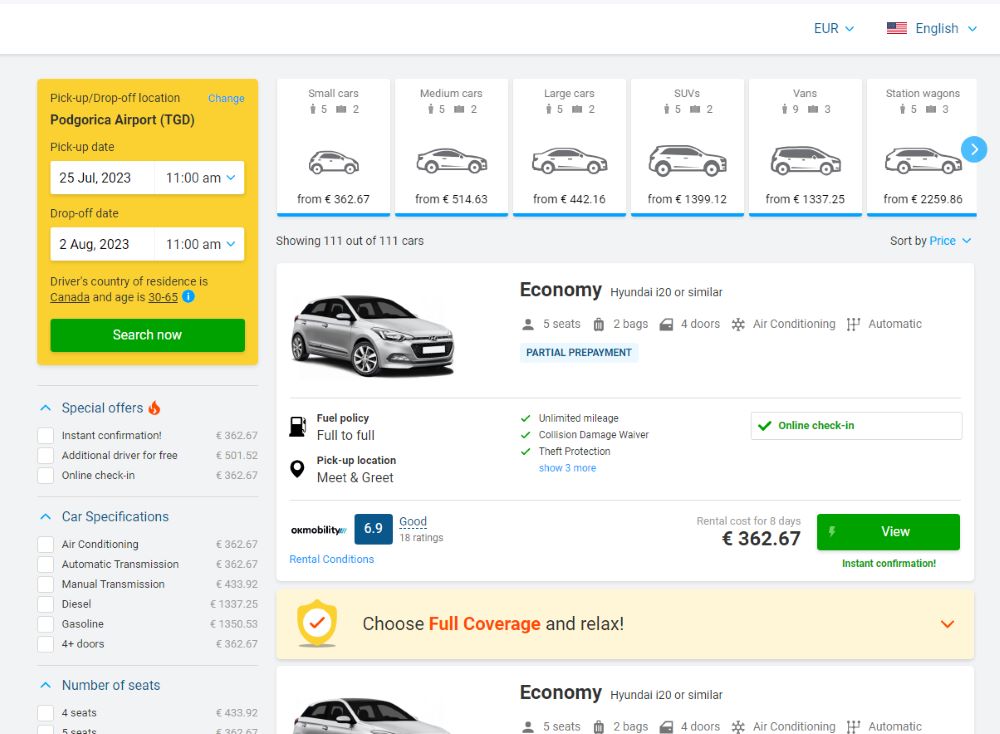### Detailed Vehicle Rental Page Description

The image depicts a comprehensive vehicle rental page with several features:

At the top of the page, users can toggle between Euro and English language options.

To the right, there's a prominent yellow box for selecting pick-up and drop-off locations, specifying pick-up and drop-off dates, and entering the driver's country of residence. Additionally within this section is a calendar feature, an age range selector (30 to 65 years), and a green "Search Now" button.

Below this box, there are promotional highlights including:
- Special Orders
- Instant Confirmation
- Additional Driver for Free
- Online Check-in

In the subsequent section, vehicle specifications are detailed:
- Air Conditioning
- Automatic Transmission
- Manual Transmission
- Diesel
- Gasoline
- 4+ Doors

Further below, seating arrangements are indicated, showing options for 4 or 5 seats. The content seems partially cut off, hinting at additional specifications not visible in the image.

At the top, six boxes are displayed horizontally, each depicting different vehicle types ranging from small cars to station wagons, arranged left to right.

The page introduces an economy vehicle option, specifically a Hyundai i20 or a similar model:
- 5 Seats
- 2 Bags
- 4 Doors
- Air Conditioning
- Automatic Transmission
- Partial Prepayment

Directly below these details, the fuel policy is outlined as “Full to Full,” and the pick-up location is designated as "Meet and Greet."

To the right, several features are highlighted with green check marks:
- Unlimited Mileage
- Collision Damage Waiver
- Theft Protection

An expandable "Show More" tab is available for additional information.

There is also a section indicating online check-in availability, marked with a green check and accompanied by green text. A rating of 6.9 (Good) based on 18 reviews is displayed. On the far right, the rental cost for 8 days is listed in Euros: €362.67, with a green "View" button adjacent to it.

Below this information, an advertisement promotes the option to "Choose Full Coverage and Relax."

Another economy Hyundai model is showcased with identical specifications to the previously mentioned car.

This detailed layout provides a clear depiction of the various options and features available for renting vehicles on the page.